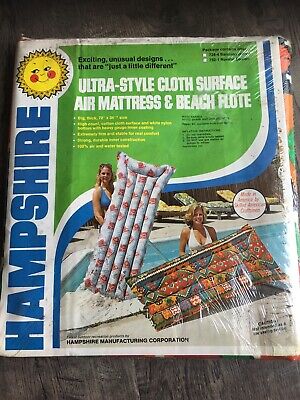The image depicts the front of a package for an air mattress and beach float, set against a backdrop of weathered, grayed wood with a dark shadow at the top. The package itself is wrapped in clear plastic and features a white background with bold design elements. On the left-hand side of the label, the word "Hampshire" is vertically inscribed in large blue letters. The top left corner showcases a cheerful, smiling sun with rosy cheeks.

Adjacent to the sun, in the upper right corner, a lime green section with black text reads, "exciting unusual designs that are just a little different." Directly below this, the main product description is prominently displayed in large, white bold letters: "Ultra Style Cloth Surface Air Mattress and Beach Flote," with "Flote" intentionally spelled with an 'E' at the end. 

The lower portion of the package features an image of two women in bikinis or swimsuits, standing by a pool and holding large, vividly designed air mattresses or pool floats. Though there are paragraphs of text in black and yellow under this image, they are too small to be legible.